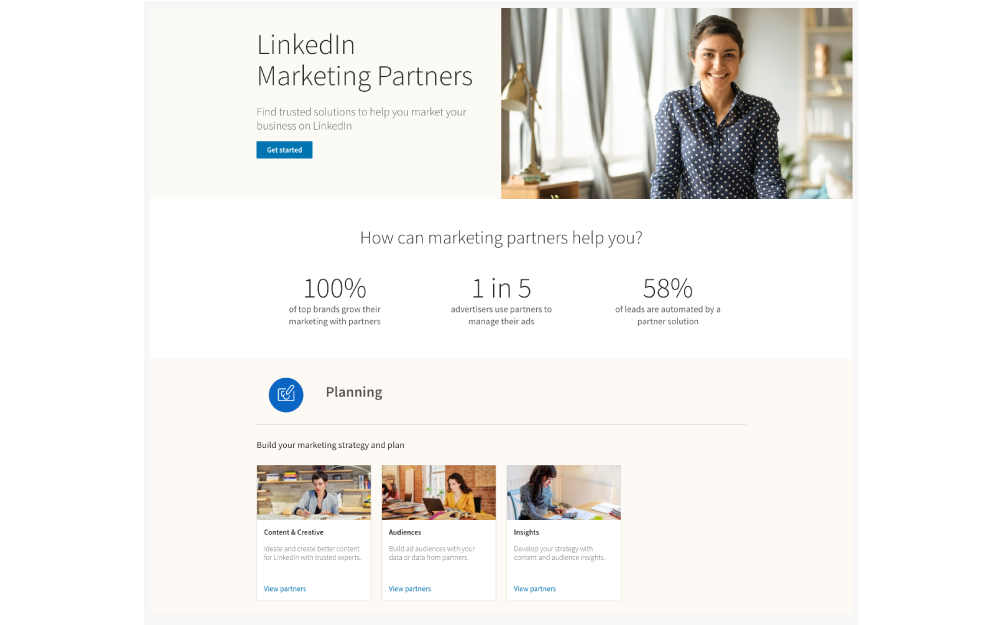The image is a detailed screenshot of a LinkedIn webpage focused on Marketing Partners.

At the top of the page, within a light gray banner occupying about a third of the page's width, the LinkedIn logo is displayed in a subtle, light gray font. Directly beneath the logo, the text "Marketing Partners" is prominently featured, followed by a smaller tagline: "Find Trusted Solutions to Help You Market Your Business on LinkedIn." To the right of this text, a blue button with white lettering invites users to "Get Started."

Accompanying the text on the right is a professional photograph of a young woman. She appears to be a white female in her 30s with very short, dark-colored hair. The woman is wearing a stylish blue and white polka dot long sleeve blouse and is smiling warmly. The background suggests she is in a well-appointed room, featuring gray curtains, white walls, a wall rack for knickknacks, and a lamp on the left side of the frame.

Below this section, a white rectangular area presents a compelling brief on the benefits of using Marketing Partners on LinkedIn. It reads:
- "How Can Marketing Partners Help You?"
- "100% of top brands grow their marketing with partners."
- "One in five advertisers use partners to manage their ads."
- "58% of leads are automated by Partner Solutions."

At the bottom of the screenshot, three smaller images are labeled "Content Creative," "Audience," and "Insight," suggesting further details about the types of services offered by LinkedIn Marketing Partners.